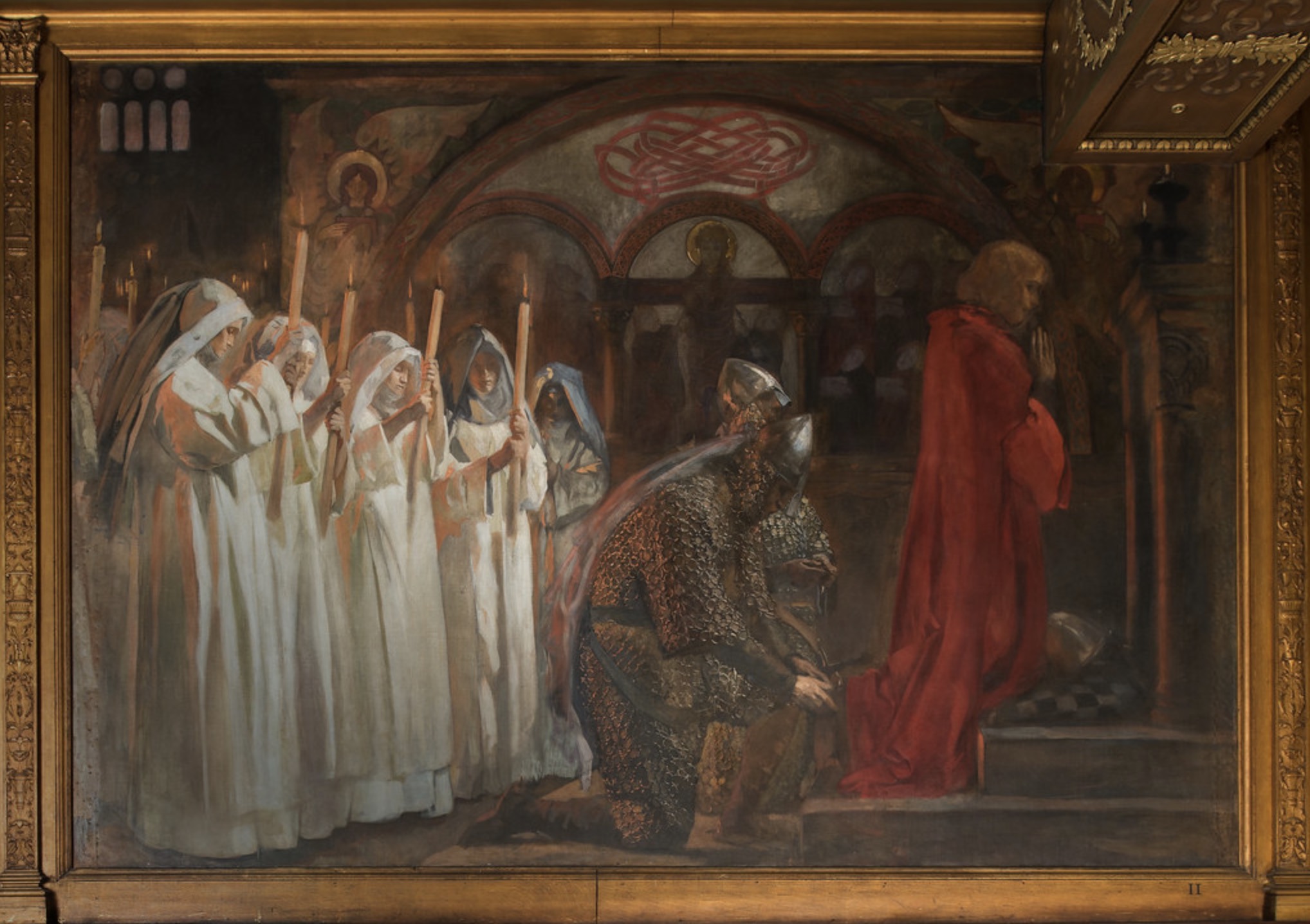This rectangular painting, encased in an ornately carved and gilded gold frame, exudes a profound religious ambiance. The scene is set in what appears to be a sacred church or temple, characterized by a striking black and white tiled area resembling a podium. Dominating the center, a red-robed figure with chin-length hair is captured kneeling in prayer, flanked by two armored men-at-arms in full chain mail and helmets. Behind this trio, forming two solemn rows, are nuns in white robes, each holding a lit, handmade, tapered candle, their expressions somber and reflective in the subdued light. The background features intricate Celtic knotwork, adding layers of historic and spiritual significance. The painting further highlights architectural elements with great detail, and in the upper right-hand corner, a protruding gold box adds an element of mystery. Despite a thorough observation, no artist's signature is visible. Overall, the artwork masterfully blends sacred iconography with meticulous architectural depiction, invoking a deep sense of reverence in the viewer.